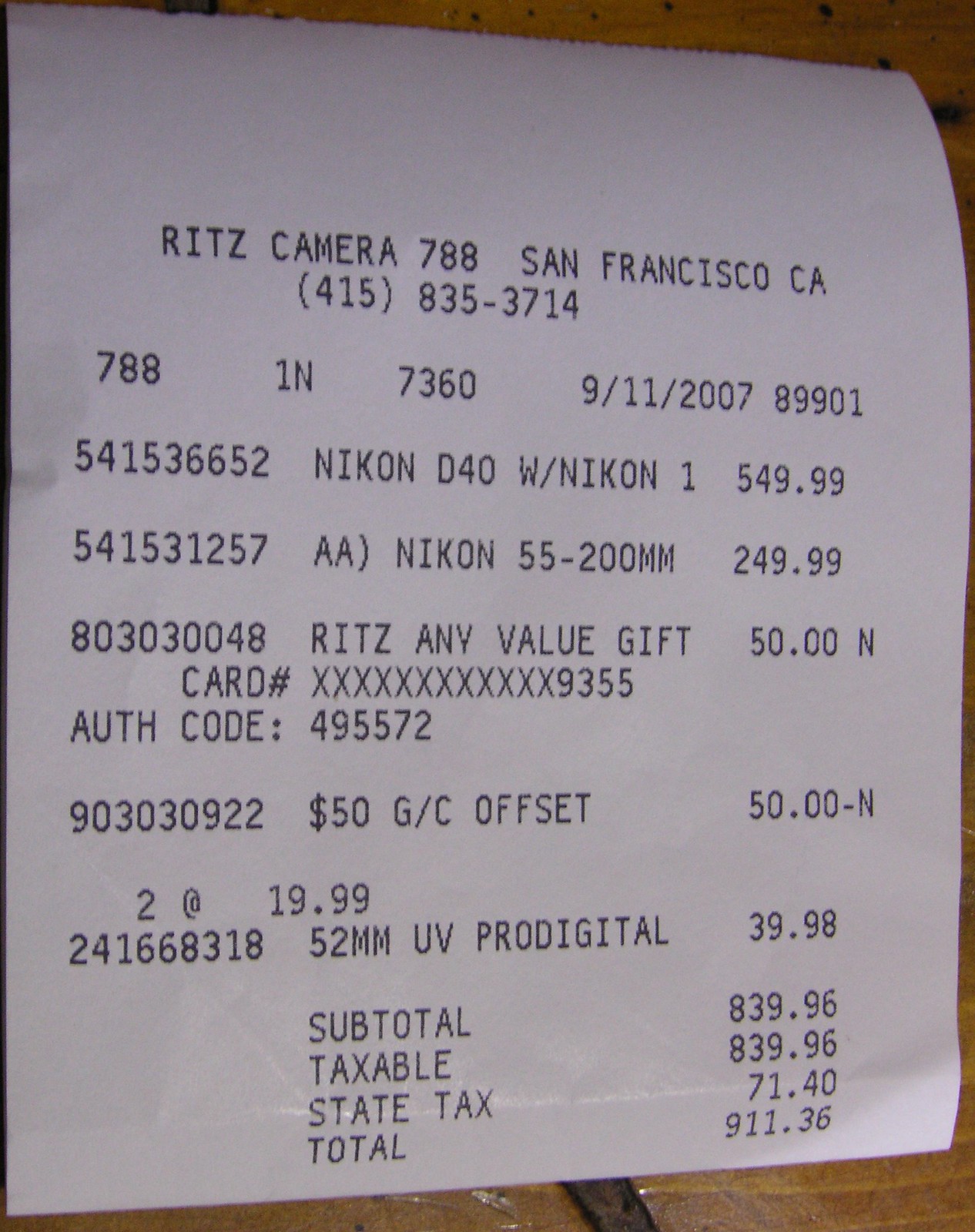The image displays a detailed receipt from Ritz Camera, located at 788 San Francisco, CA, with the phone number 415-835-3714. The receipt is dated September 11, 2007. Below are the listed items purchased:

1. Nikon D40 with Nikon 1 accessory for $549.99.
2. Nikon 55-200mm lens for $249.99.
3. Ritz AnyValue gift card, ending in 9355, valued at $50.
4. $50 gift card offset.
5. UV ProDigital filter for $39.98.

The subtotal before tax is $839.96. After adding state tax, the total comes to $911.36. The receipt is printed on white paper with black text.